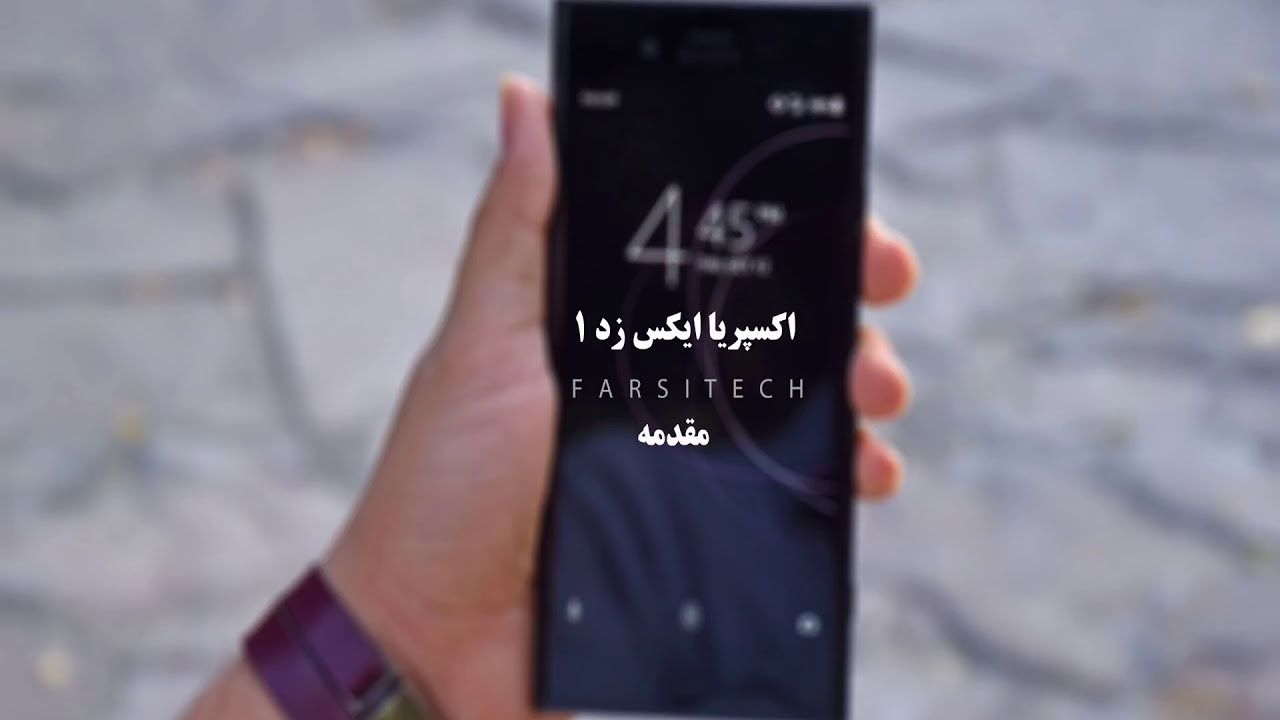The image is a color photograph in landscape orientation, likely for an advertisement, showing an extreme close-up of a man's left hand clutching a black rectangular cell phone. The hand dominates the view, with the thumb to the left and three other fingers visible to the right. The phone screen, facing the viewer, displays a barely legible digital clock at the top and some icons near the bottom. Overlaid on the screen are three lines of white text in a foreign language, with the word "Farsitech" prominently featured in the center. The hand also reveals a brownish-purple leather watch band around the wrist. The blurry background shows a cracked, bluish-grey concrete ground, giving a textured effect to the otherwise minimalist setup. The graphic design typography combines with the photographic imagery to create a stylized, representational advertisement.